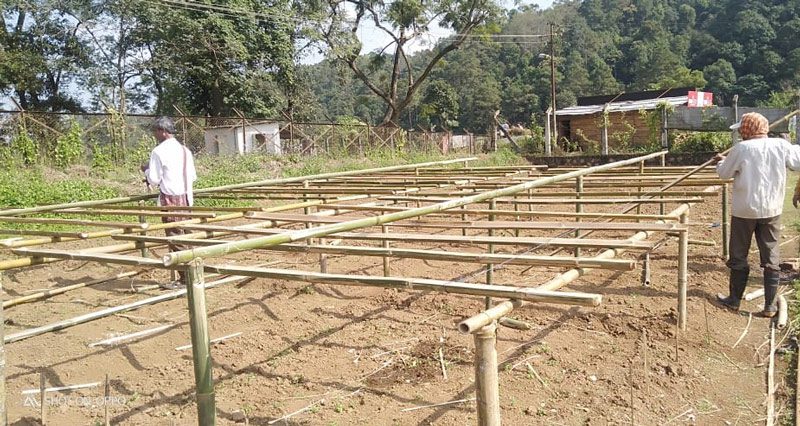In this color photograph taken outdoors, two construction workers are diligently crafting a bamboo structure within a tilled, bare-earth setting reminiscent of a garden or farm. The workers, both seen from the back, are placing bamboo posts into the ground, forming a grid-like pattern. The structure appears to be approximately three feet high and spans an estimated 10 by 20 feet. The worker on the left, wearing a white shirt and brown pants, has a darker complexion and gray hair, while the worker on the right sports a white jacket, gray pants, and a hat with an orange and black scarf. He is seen holding a long wooden stick. Surrounding them is thick greenery with trees, shrubs, and grasses, and there's a hint of a blue and white sky visible through the forest. In the background, dilapidated outbuildings with indistinct signage and a wooden fence blend into the scene. A telephone line runs off to the side, adding to the rustic ambiance. The exact purpose of the bamboo construction is unclear, but it might serve as an elevated flooring or a framework to shade crops.